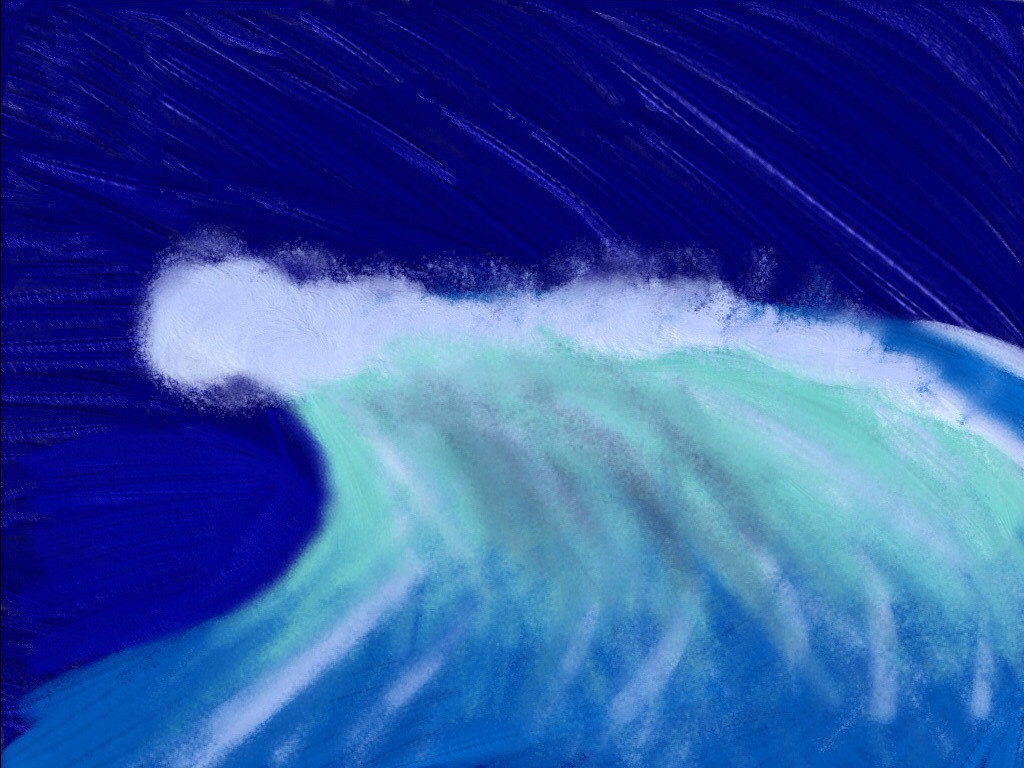This image depicts a striking piece of artwork featuring a powerful ocean wave. The artwork exudes a lifelike depth through meticulous brushstrokes or digital strokes that mimic the texture of acrylic paint on canvas. Dominated by a background of dark blue, interspersed with horizontal streaks of lighter blue to represent the vast, churning sea, the wave dramatically arcs from the bottom left towards the top right in a graceful c-shaped curve. Cresting at the peak, the wave showcases its turbulent nature with frothy, white foam that has been skillfully smudged to simulate the spray of the ocean. The wave transitions through a captivating spectrum of colors, starting with white at the crest, blending into a greenish-teal and bluish hues, and deepening into darker blue towards the wave’s base. This dynamic composition captures the raw beauty and movement of an ocean wave breaking, demonstrating an impressive blend of color and texture that immerses the viewer in the scene.